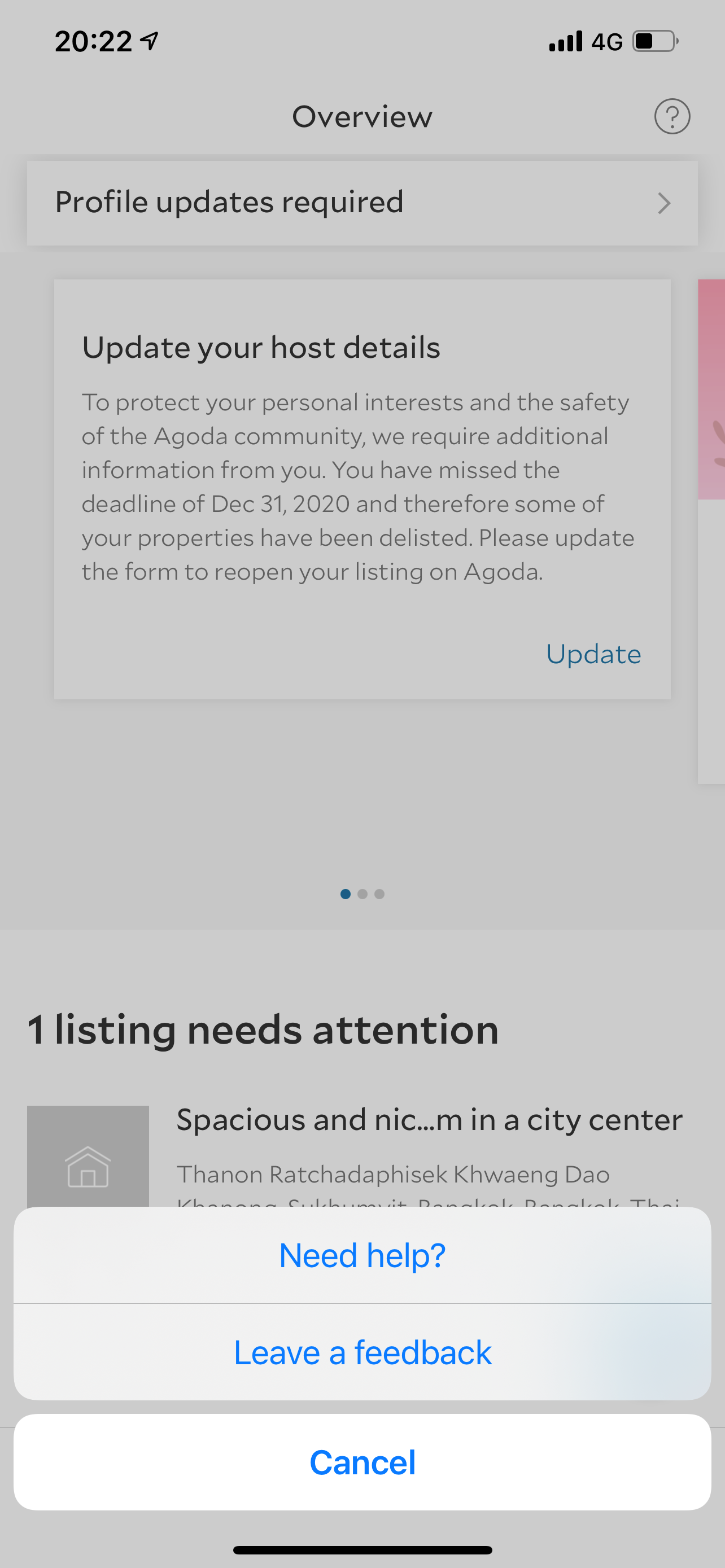**Detailed Caption:**

This image is a detailed screenshot from a smartphone displaying the customer interface of the Agoda app. The phone is set to military time, showing the time as 20:22 (8:22 PM). The device has strong connectivity with full 4G signal and a partially drained battery at approximately one-third capacity.

The focal point of the screenshot is the "Overview" page of the Agoda app, indicated by a bold "Overview" title with a question mark symbol next to it. The page displays an alert message stating that "Profile updates are required." An arrow icon accompanies this notification.

Beneath this heading, a detailed message informs the user that they need to "Update your host details." The text specifies that to protect personal interests and maintain the safety of the Agoda community, the app requires additional information. It notes that the user missed the December 31, 2020, deadline for these updates, leading to the delisting of some properties. Users are prompted to complete the required form to reinstate their listings on Agoda. A prominent blue "Update" button is positioned below this message.

At the interface's bottom, three small dots suggest a multi-page format, with the first dot highlighted in blue, indicating the current page. Below the main message, there's an alert caption stating, "1 listing needs attention," followed by the partially visible listing name: "Spacious and nice... in a city center," specifying the city where the listing is located.

Towards the bottom, three interactive buttons are available for user action: "Need help," "Leave feedback," and "Cancel." The first two buttons ("Need help" and "Leave feedback") are set against a gradient gray background, while the "Cancel" button has a white background.